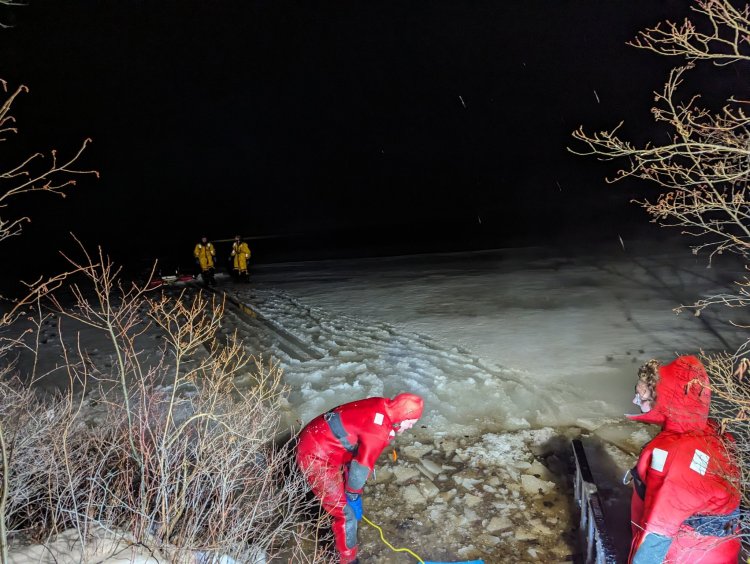In this color photograph set during the evening, a group of people is gathered on and beside a frozen body of water under a pitch-black sky. The foreground reveals two men in red coveralls with hoods; one is visible from the waist up, standing to the right, while the other is bent over, closely examining something on the ground, possibly a yellow wire. Footprints lead across the snow-covered surface towards two figures in yellow raincoats standing at the edge of the water, facing the shore. The scene is framed by leafless trees and shrubs on both sides, indicating wintertime, and there is a noticeable red and white object near the people in yellow coats. The ground nearby features patches of dirt or old seaweed, adding to the desolate, wintry feel of the landscape.